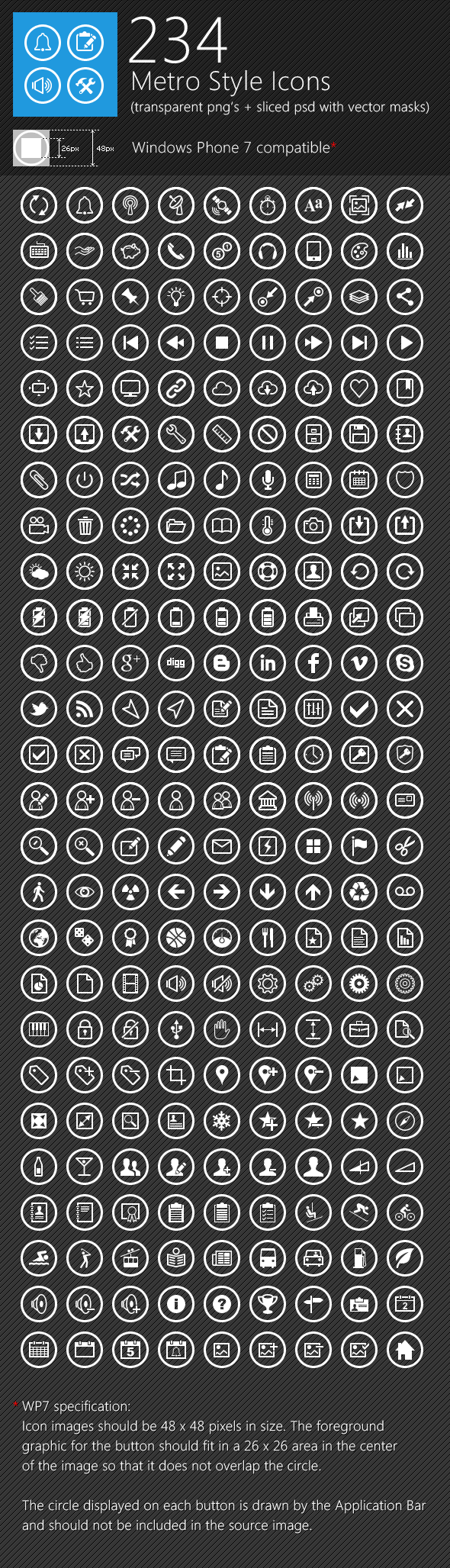**Detailed Description:**

The image in question is a vertically oriented, rectangular digital file that is significantly taller than it is wide. It features a predominately black background with white text, creating a high-contrast visual effect that is easy to read. 

At the top-center of the image, the text "234" is displayed prominently. To the top-left corner, there is a blue rectangular box containing four icons, each enclosed within a circle. The icons represent different functions: volume control, tools, an alert, and one that resembles a clipboard.

Beneath the initial "234" label, the text "Metro style icons" is centrally positioned, followed by the phrase "(transparent PNGs + slice PSD with vector marks)" in parentheses. Further down, still centrally aligned, the text "Windows Phone 7 compatible" appears with a red asterisk beside it.

There is a symbol resembling "26PX, 49PX" situated below, indicating pixel dimensions, which is likely a reference to the size of the icons or images.

The core of the image consists of a grid layout that showcases rows of circular icons, each row containing nine icons. There are approximately 30 or more such rows, indicating a vast collection of over 270 distinct icons. The icons cover a wide array of functionalities — the first row includes icons for alerts, satellites, and alarm clocks. The second row features icons such as keyboards, phones, and headsets. Each icon maintains a uniform design style consistent with the Metro iconography.

Towards the bottom, additional text seems to provide further details or descriptions, potentially highlighting the extensive variety of icons available, although the precise applications or target audience of the icons remain unclear.

Overall, the image serves as a detailed catalog or sample sheet of Metro-style icons, meticulously organized and compatible with Windows Phone 7, aimed at designers or developers in need of high-quality, versatile iconography.